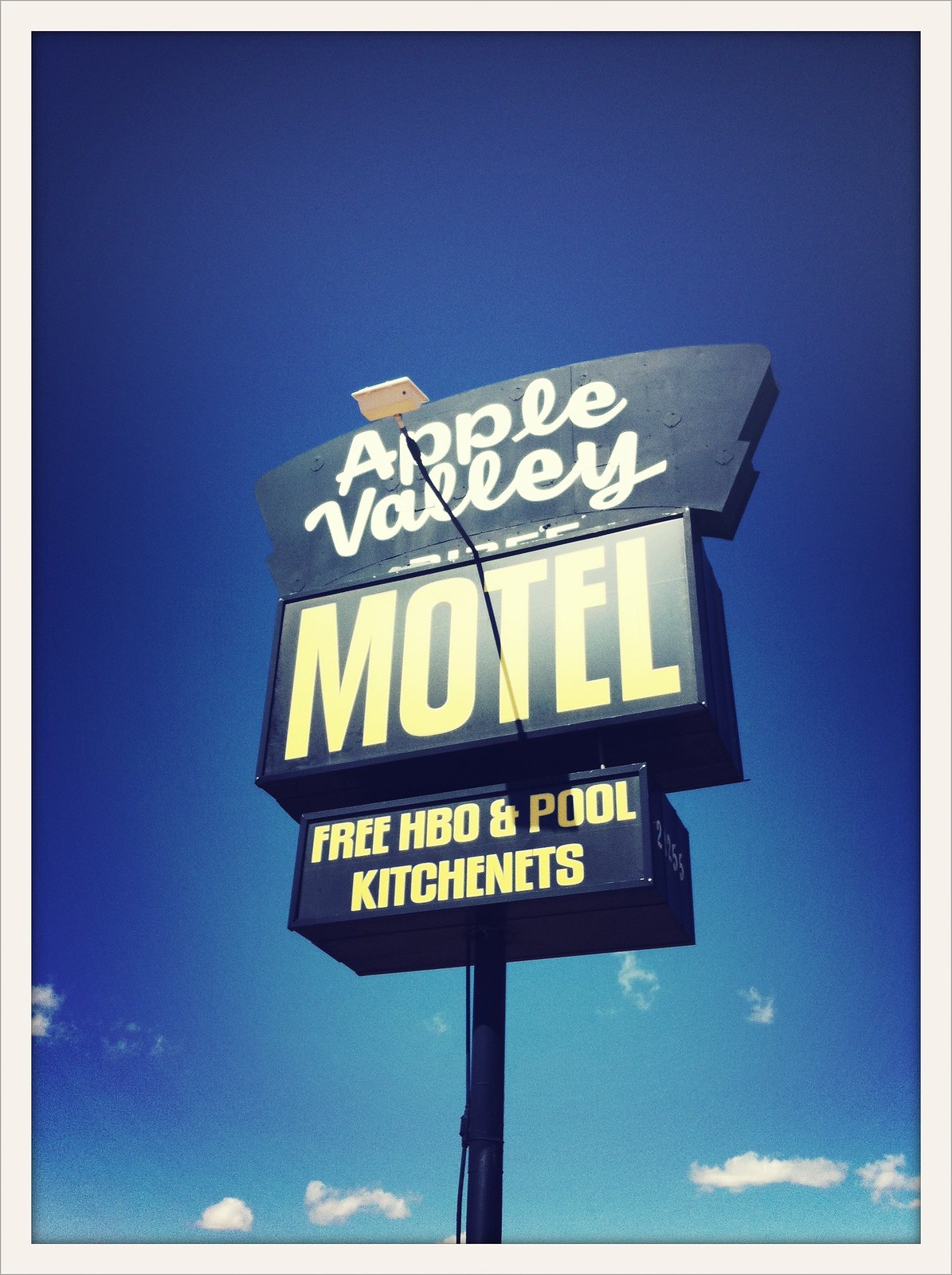The image features a large roadside sign perched on a substantial black pole. The sign prominently displays "Apple Valley" at the top, with "Motel" directly below it. Beneath "Motel," it advertises amenities including "Free HBO and Pool Kitchenettes." 

The sign, which appears blue with yellow lettering, stands out clearly against a vibrant blue sky dotted with fluffy white clouds. There are no other discernible objects in the image, allowing the viewer’s focus to remain solely on the brightly lit, well-maintained sign. The background sky transitions from a lighter blue near the horizon to a deeper blue as it stretches upwards. The overall scene is bathed in natural light, providing excellent clarity and a bright, vivid setting.